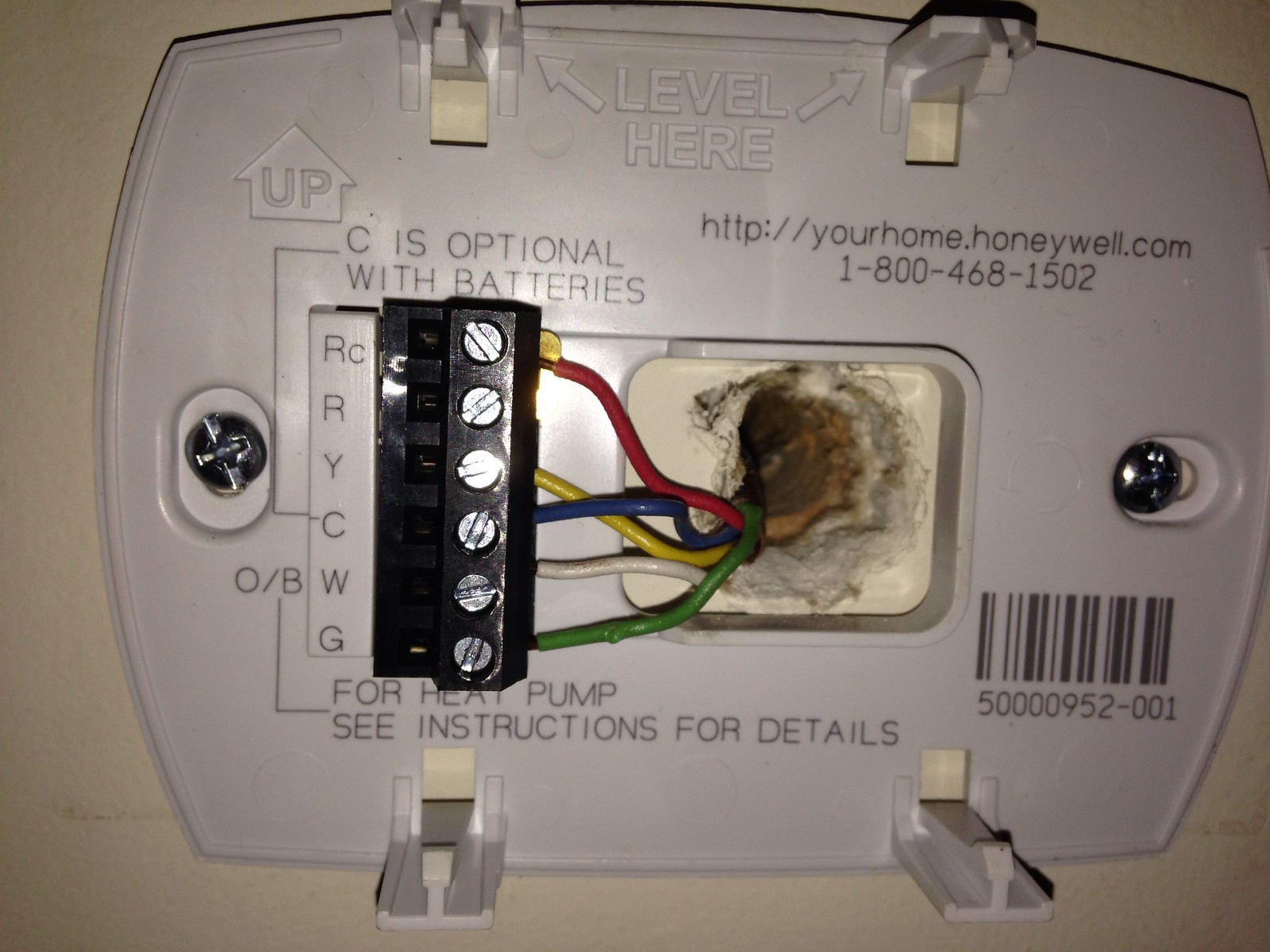This photograph captures a close-up view of a white plastic plate mounted on an off-white (slightly yellowed) wall. The wall forms the backdrop and is visible in all four corners of the image. The plastic plate prominently features various imprinted labels and information.

At the top of the plate, the words "Level Here" are inscribed with two arrows pointing left and right towards small mounting notches. Just below this, an arrow labeled "Up" is imprinted in the center with a web address "http://yourhome.honeywell.com" in black font placed beside it. Beneath the web address, the phone number "1-800-468-1502" is clearly visible.

Further down, under the "Up" arrow, the words "C is optional with batteries" are stated. Following this text is a vertical line with the labels "RC," "R," "Y," "C," "W," and "G" listed in order. Adjacent to these labels, "O/B" is indicated with a downward arrow next to it, along with an instruction "For heat pump, see instructions for details."

In the center of the plastic plate, there is a hole revealing four distinct colored wires protruding from the wall, ending in a small metal piece with a black tip. This detailed and informative arrangement suggests that the plastic plate is part of a Honeywell thermostat mounting system, providing clear guidelines for installation and wiring.